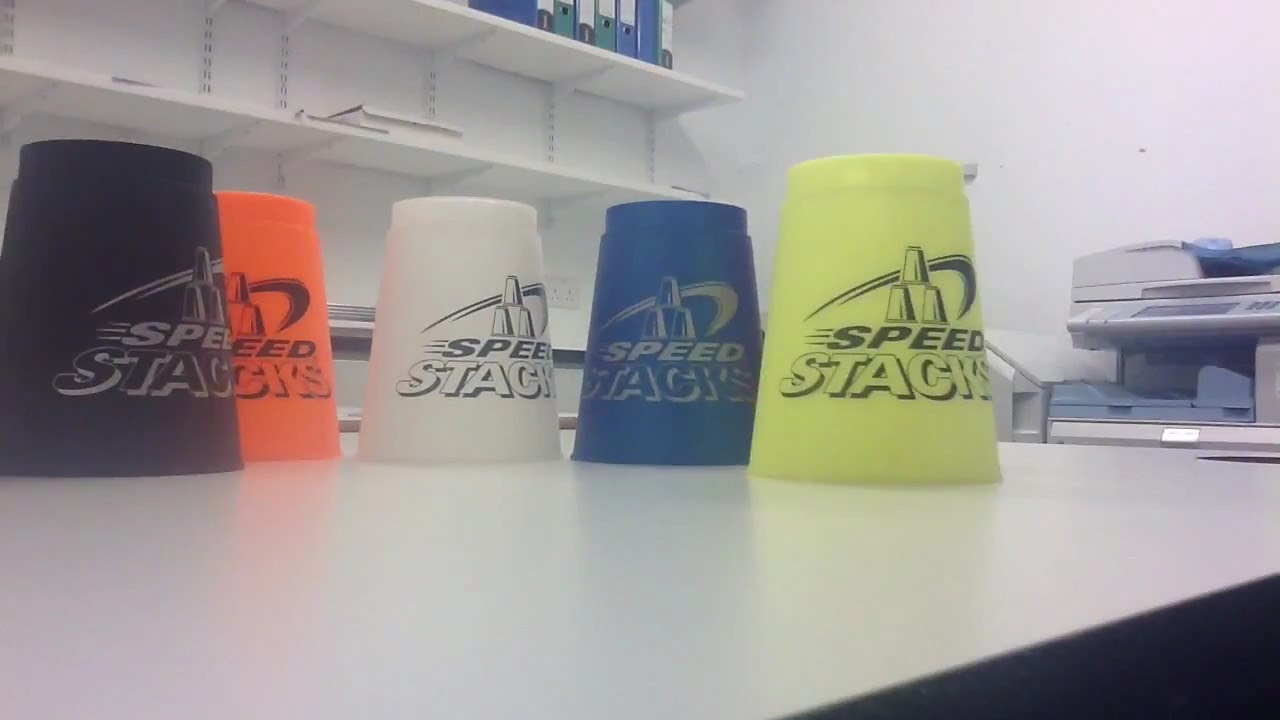This color photograph, oriented in landscape, captures a white table surface at close range, with five upside-down plastic cups prominently displayed in a rounded formation. Each cup bears the "Speed Stacks" logo, which depicts three inverted cups arranged in a pyramid with a swirling background. The cups are positioned almost centrally, spanning two-thirds of the way across the image. Their colors from left to right are black, orange, white, blue, and a vibrant yellow, with the yellow cup appearing the closest and largest due to the perspective. In the background, the upper left corner features white shelves with visible blue and green binders atop, while a gray printer is situated on the middle right side, suggesting an indoor office or competitive stacking setting.